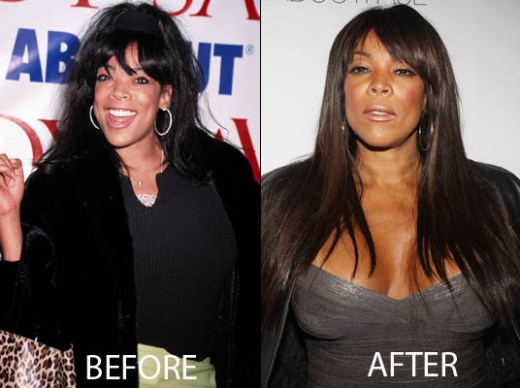The image is a collage of before and after photographs showing the same woman. On the left side, the "before" picture depicts the woman wearing a dark top and large hoop earrings, smiling broadly. She stands in front of a backdrop with red and blue lettering on a white background. Her hair is shorter, and she is holding a white leopard skin patterned bag. On the right side, the "after" picture shows the woman in a very low-cut, grey top, with her hair much longer and appearing tanned or amber. She wears big hoop earrings and smiles, albeit less broadly, in front of a solid white backdrop. The words "before" and "after" are positioned at the bottom left and bottom right of the image, respectively.